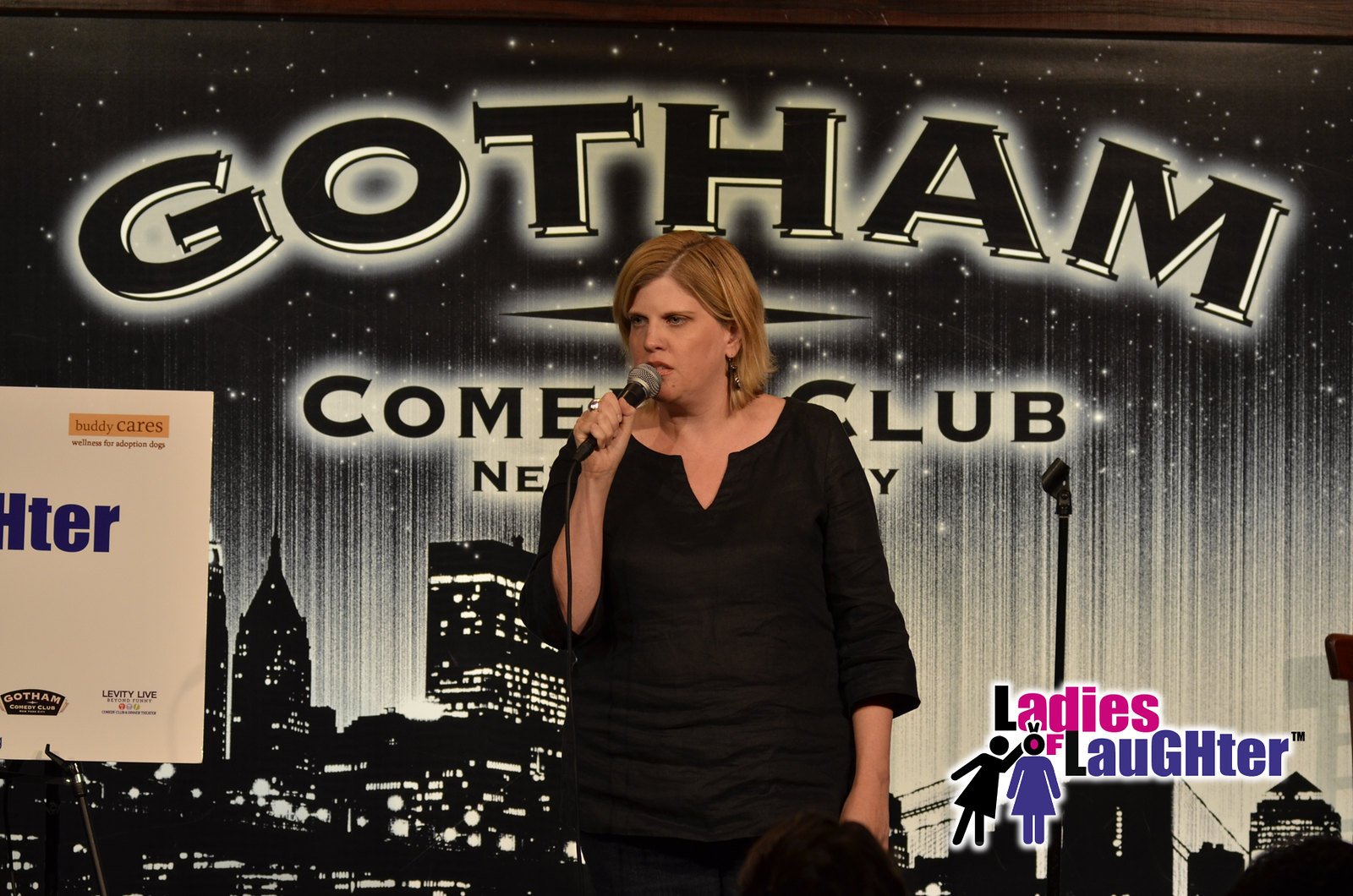In this photograph, a woman with medium-length ginger red hair and a black outfit is performing stand-up comedy, holding a black microphone. Her ensemble includes a black blouse with an open top and black pants, with one hand casually placed in her pocket. The backdrop behind her features a black-and-white design that prominently displays the "Gotham Comedy Club, New York" logo in bold Gothic font. The background also depicts a silhouetted New York City skyline with illuminated windows and a starry night sky above. In the lower right corner, the text "Ladies of Laughter" appears alongside cartoonish images of two women – one in black and the other in blue – with the woman in black seemingly making a playful gesture toward the other.